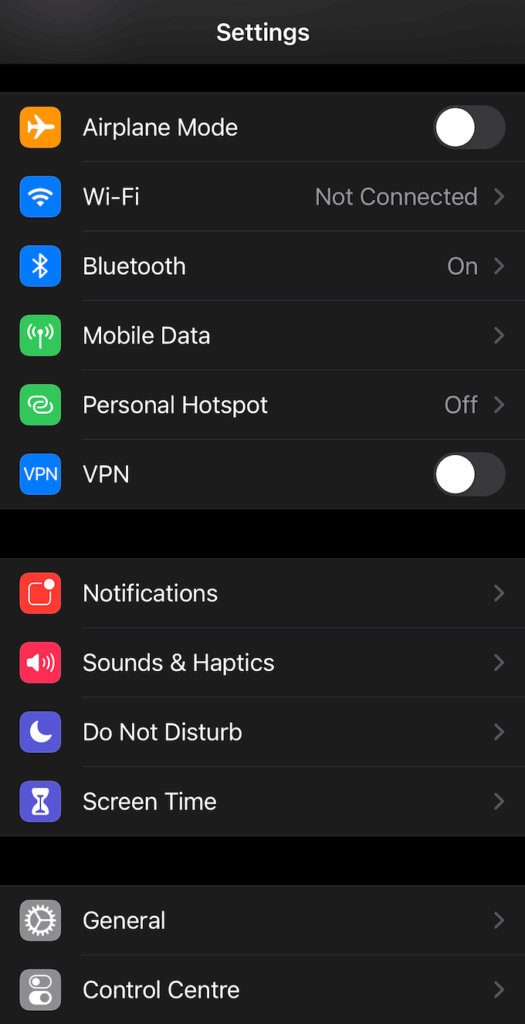Here is a detailed and cleaned-up caption for the given image:

---

The screenshot displays the settings interface with a black background. On the left side, there are rounded-square icons representing each setting, while the right side shows the status of these settings. 

Specifically:
- **Airplane Mode**: Enabled, with the slider positioned to the left.
- **Wi-Fi**: Not connected.
- **Bluetooth**: Enabled, indicated by the slider on the right.
- **Mobile Data**: Off.
- **Personal Hotspot**: Off.
- **VPN**: Enabled, with the slider set to the left.

The sections are color-coded in a lighter gray:
- The settings from Airplane Mode to VPN are in one shade of lighter gray.
- The settings from Notifications to Screen Time are in another shade of lighter gray.
- Lastly, the General and Control Center settings are also in a lighter gray.

This structured layout provides a clear overview of the user's current settings and their respective statuses.